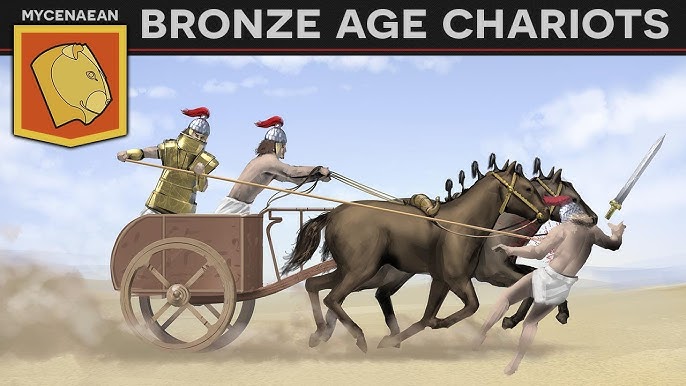The image is a digital depiction set outdoors, featuring a Mycenaean Bronze Age chariot scene. At the top, a black banner with white text reads "Mycenaean Bronze Age Chariots", accompanied by a yellow, red, and black logo with an animal head underneath the name "Mycenaean". In the scene below, two brown horses draw a brown chariot with large tannish wheels, ridden by two men dressed as Roman gladiators. One man is adorned in gold armor with metal shields covering his wrists and body, and a silver helmet topped with red feathers. The other man is shirtless, wearing white pants and a silver helmet with red feathers. The background features a clear blue sky dotted with clouds. In the foreground, a man dressed in a white loincloth, holding a sword, appears to be knocked over by the horses, as dust rises from the sandy desert-like ground beneath them.